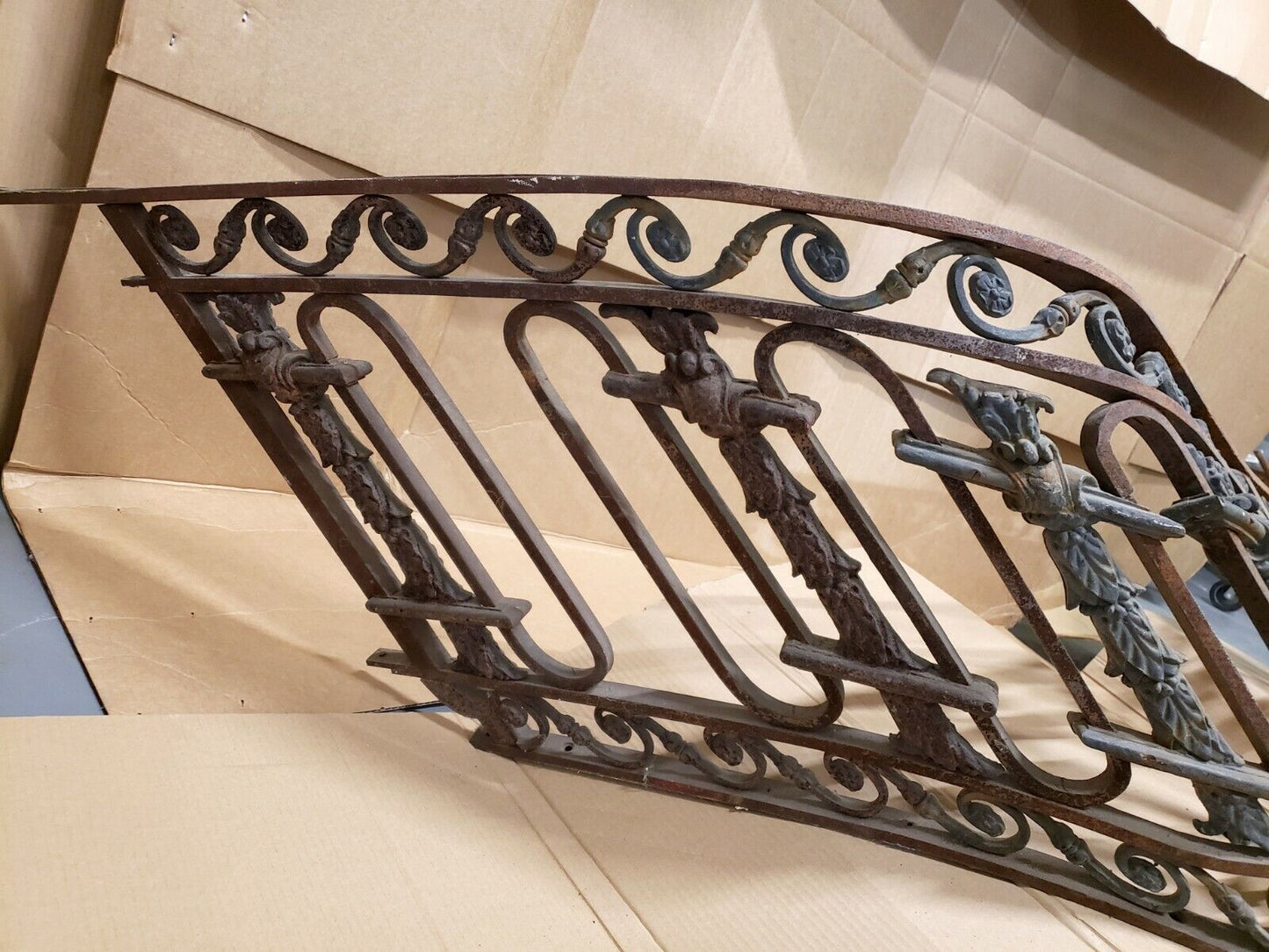This photograph depicts a distorted or warped image of an ornate metal gate resting against a backdrop of flattened, multi-layered cardboard. The gate, seemingly made of iron and almost rust-colored, features intricate designs including wavy bars, swirl patterns, and alternating leafy designs interspersed with circle oval loops. The image distortion makes the gate appear bent and tilted to the left. The metal structure lies on and is surrounded by unwrapped cardboard surfaces, some of which are positioned on the ground while others lean against a background wall, enhancing the scene's sense of disarray.